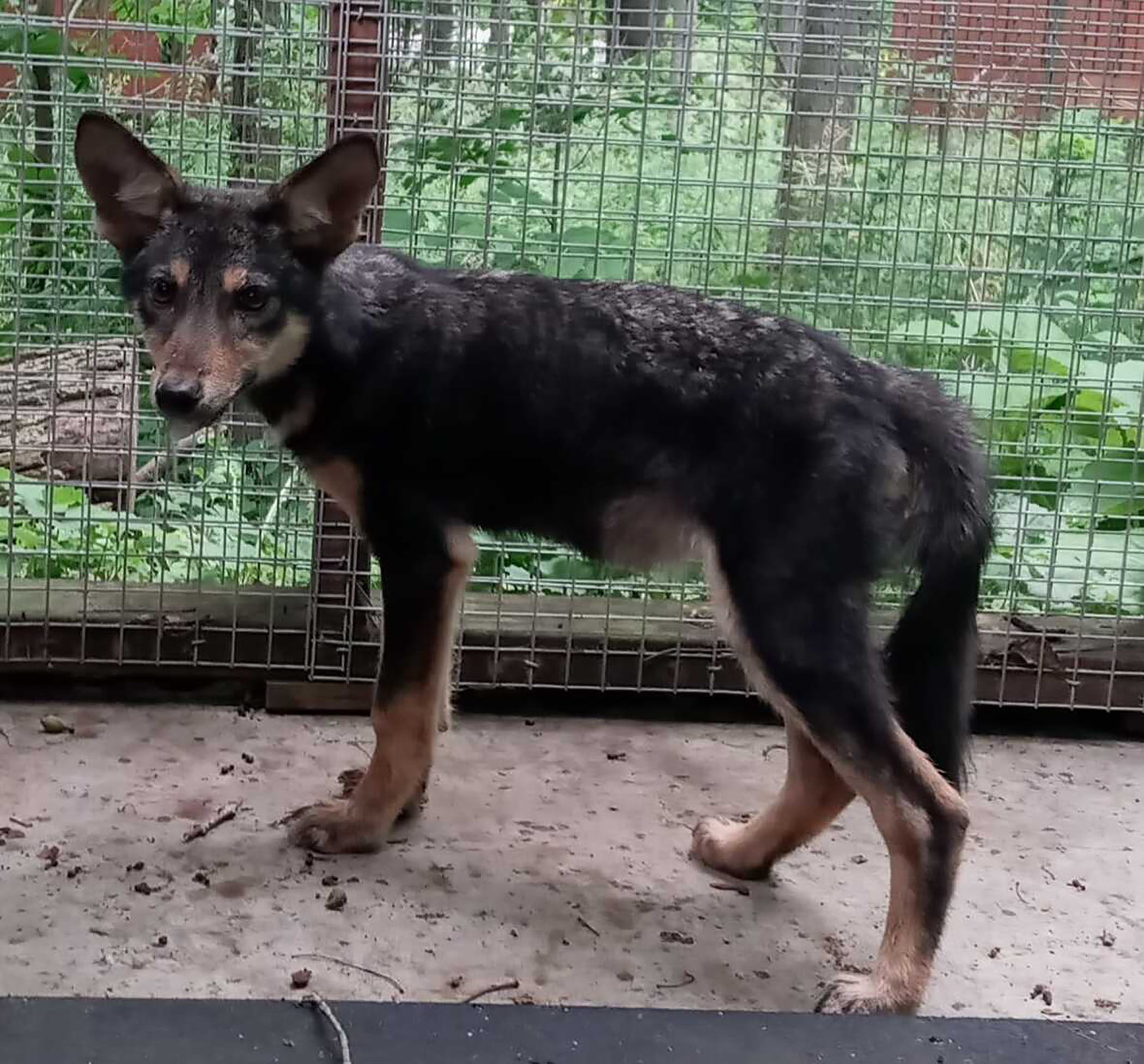The photograph showcases a sorrowful, medium-sized dog confined within an outdoor shelter kennel. The dog appears emaciated and unhealthy, with its tail tucked between its legs and a sad expression on its face. Its predominantly black fur is complemented by patches of brown above its eyes, on its legs, and hints of gray and white along its back and tail. The dog's large, triangular ears stand erect, its head turned towards the camera, while its body faces to the left. The dog stands on a rectangular patch of light gray or beige sand, enclosed by a double-layered metal fence with square holes, supported by wooden posts. Behind this cage, the scene extends into a wooded area filled with thick, green foliage and tree trunks.